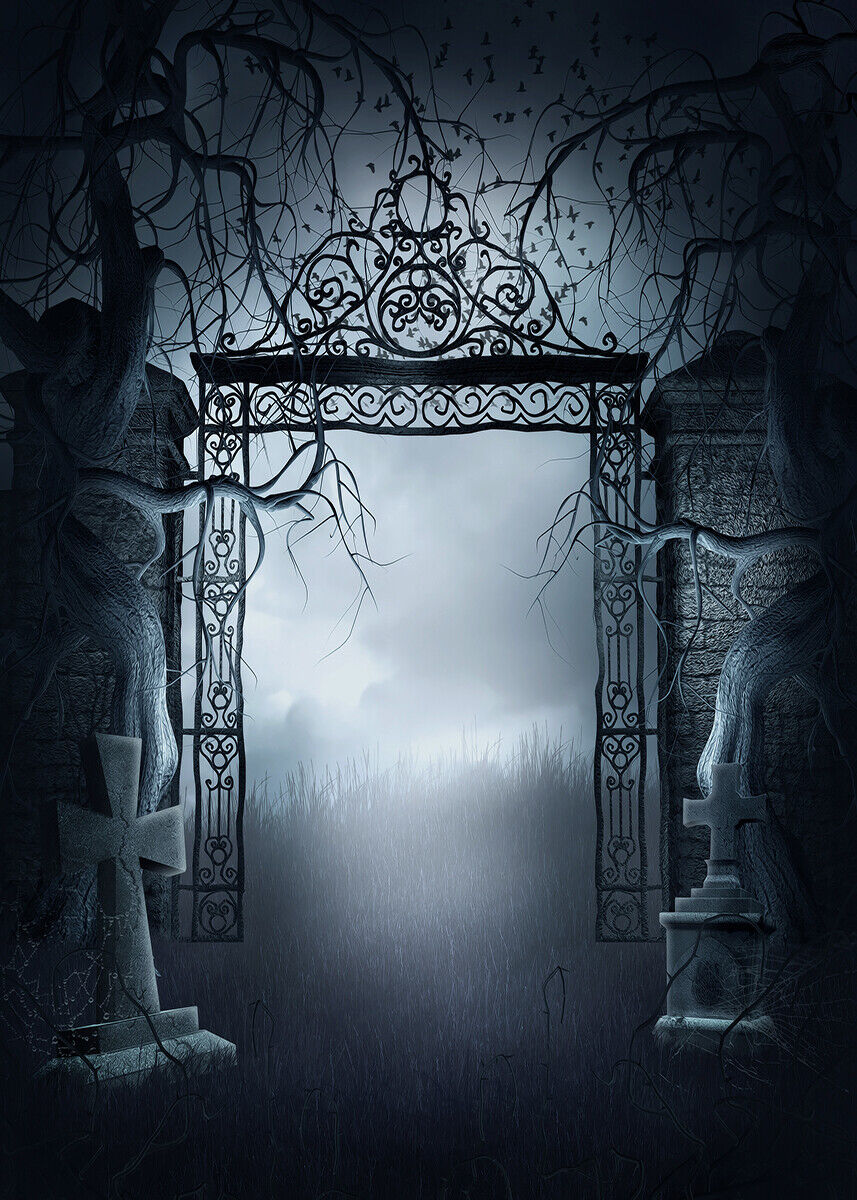The image is an AI-generated illustration with an eerie, horror-movie feel characterized by a bluish-gray tone. Depicting the entrance to a graveyard, the view appears to be from within, looking outward into a foggy, ominous forest. Centered in the illustration is a wrought iron gate, devoid of its actual gate but framed by intricate iron curls, some forming heart shapes, and twisted ironwork at the top resembling a sun. This portal connects to stone walls on either side. Leaning against these stone structures are two tombstones shaped like crosses, with another set of tombstones and dead, leafless trees further adding to the macabre atmosphere. Creeping over the arch of the gate are sinister vines, and tall, overgrown grass leads through the gate. The scene is shrouded in dark, foreboding clouds, and black birds, possibly ravens, hover menacingly in the background, enhancing the overall eerie and scary ambiance of the scene.